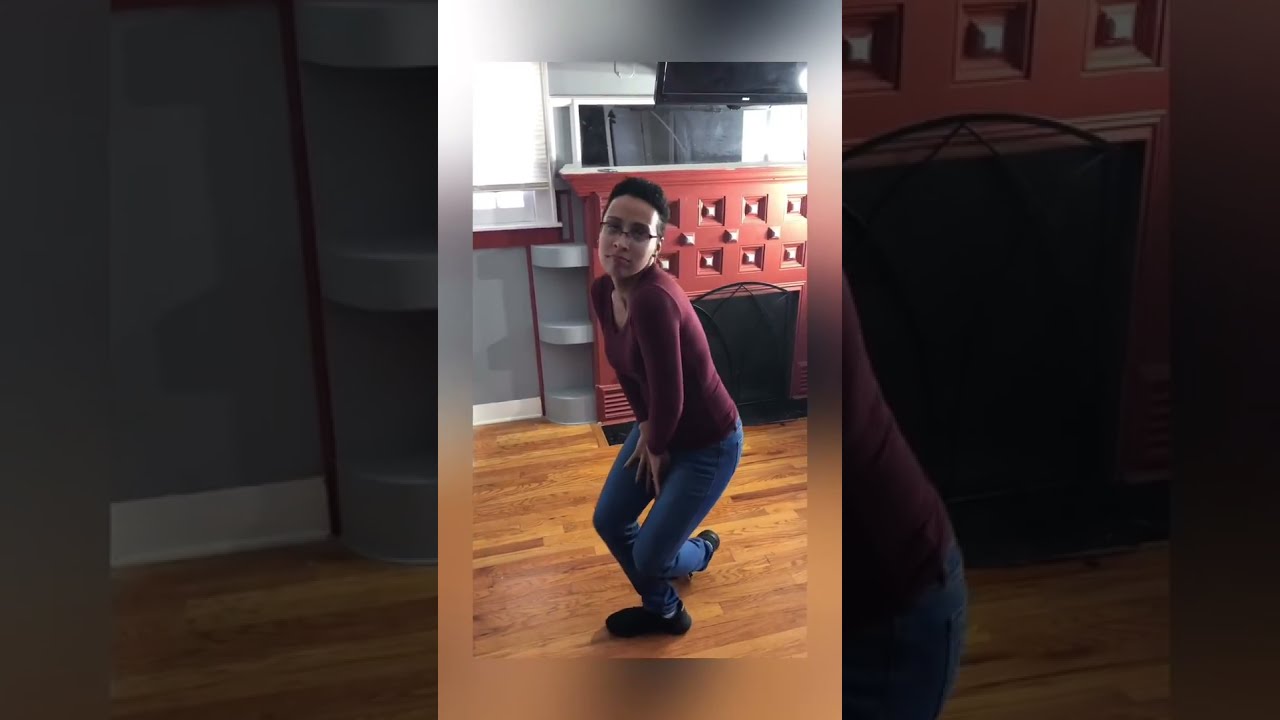In this vertical cell phone-style image, centered amidst large black rectangles on either side, we see a detailed view of a living room featuring a wooden floor. The focal point is an African-American woman with short black hair and prescription glasses, standing in a poised stance with one foot in front of the other, her left side facing the camera and her right side facing a red-colored fireplace. She wears a tight, maroon long-sleeved shirt, blue denim jeans, and tennis shoes. One of her arms is held back behind her. Above the fireplace, which has black grills and a mantle with vents and white-handled indentations, a flat-screen black TV is mounted on the wall, slightly angled downward. A light from a lamp in front of the TV shines towards the back of the woman, creating a reflective gleam on a mirror positioned below the TV. The room is illuminated further by a glare from white blinds pulled upwards on a light blue wall to the right. The flooring is a nicely varnished light hardwood. The composition of the image is such that it blurs the outer edges, emphasizing the scene within the center rectangle.